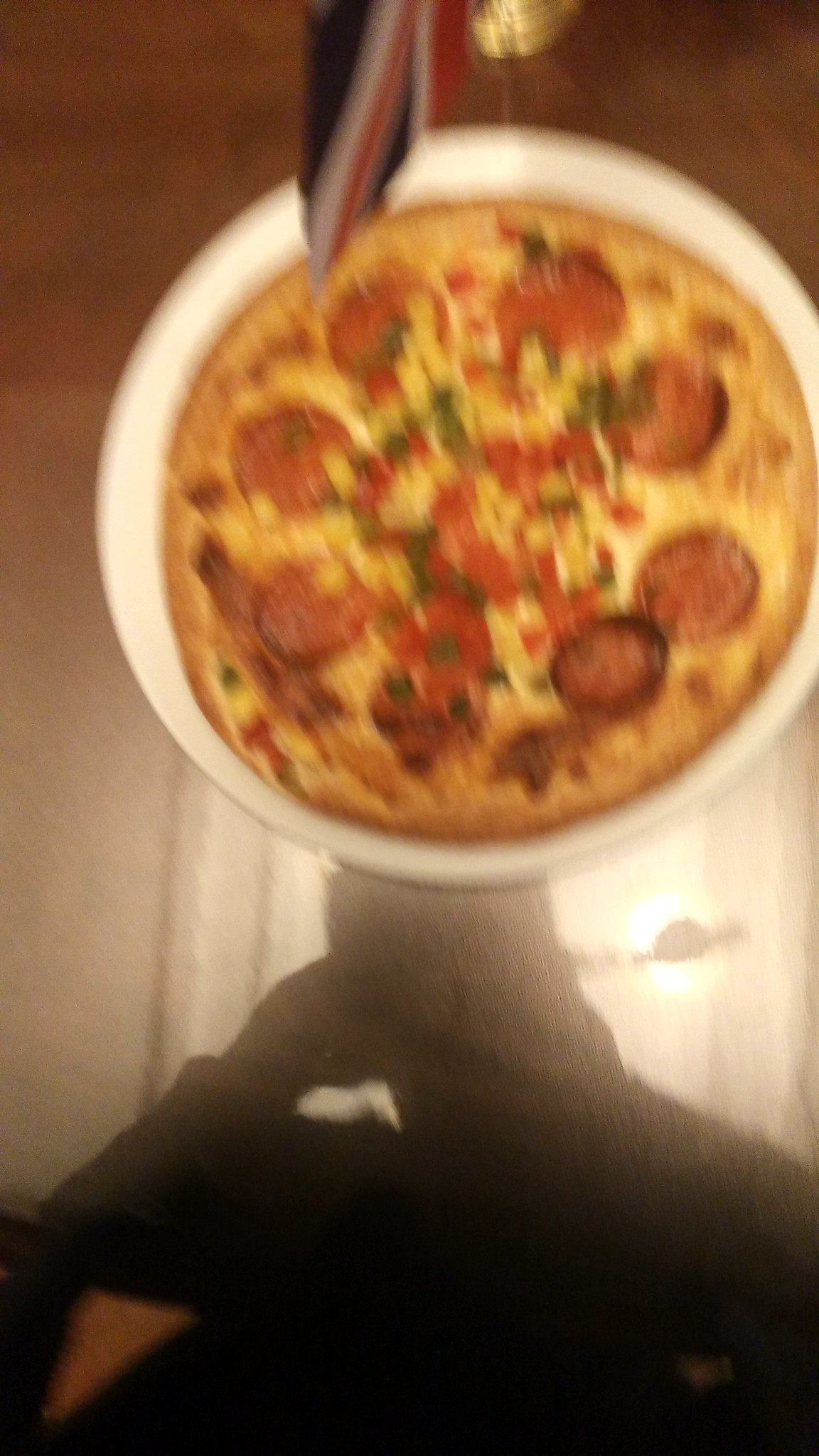The image captures a hastily taken and blurry photograph of a fresh, homemade pizza placed on a white plate atop a wooden table. The pizza, with a visibly browned crust, is topped with cheese, pepperoni, and bits of red and green bell peppers. Surrounding the pizza is a scene suggesting homeliness with the soft, warm tones of the wooden table. A British flag, implied by the partial yet recognizable Union Jack colors, is visible just off the edge of the table. A shadow, most likely belonging to the person taking the photograph, looms over the pizza, casting a dark silhouette that obscures their facial features. The harsh illumination from a light source above heightens the contrast and adds to the overall blurriness of the image. Some detailed elements, such as the glossy texture of the table and the person's black shirt, indicate the photo was spontaneously taken, focusing more on capturing the moment rather than perfect clarity.